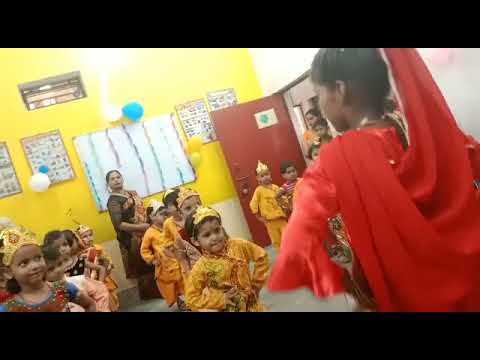The image depicts a lively and colorful scene inside a South Asian classroom, likely from India or a similar region, characterized by its cultural richness and traditional attire. The room features yellow walls adorned with various educational posters, charts, and a whiteboard, while the lower portion of the walls is white. There is a red door, partially open, with a few individuals peeking through.

Centered in the scene are numerous children, arranged in rows and wearing elaborate traditional costumes. Many of them are dressed in yellow outfits, long-sleeved with red accents, and adorned with gold hats or tiaras. The children appear engaged in a synchronized dance routine, standing with their hands on their hips, all facing the front of the classroom.

In the foreground on the right side, there is a woman dressed in a flowing red garment with cape-like elements, her back to the camera, seemingly guiding the children's dance movements. Her hair is dark and pulled up, adding to the elegance of her attire. She is contrasted by another woman on the left end of the classroom, who faces forward, clad in a black dress with a goldish scarf draped over her shoulder.

The detailed traditional attire, combined with the vibrant classroom setting, creates a vivid tableau of cultural education and joyous activity.